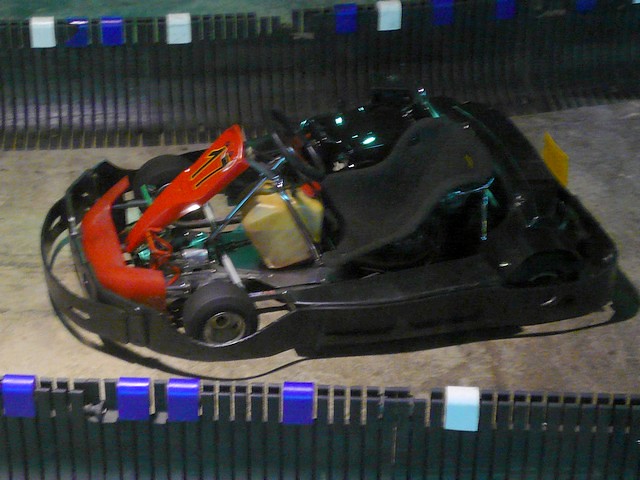The image depicts a go-kart positioned at the center of a track, potentially indicating a go-kart racing environment. The go-kart, distinguished by its basic design, features a red front marked with the number 17 and a black metal bumper that wraps around the entire vehicle for protection. The seating area includes a black chair, and there appears to be a bag or similar object placed on it. The surrounding track is composed of concrete flooring, reminiscent of a basement or standard racetrack material. Enveloping the scene is a metal fence, which is notable for its black color interspersed with white and blue stickers. The backdrop, possibly depicting an indoor or nighttime outdoor setting, completes the racing atmosphere. No people or additional text are visible beyond the number on the go-kart. The colors evident in the image include green, blue, white, tan, gray, red, green, and black.